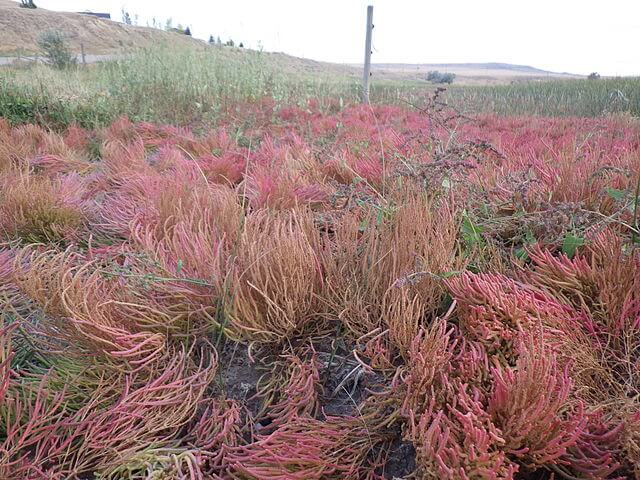The image features an expansive grass field stretching across the landscape, drenched in natural light. The foreground showcases unusual pink tufts of grass that evoke the appearance of delicate coral, peppered with hints of light brown and green. This curious flora contrasts sharply with the dominant green hue of the surrounding grasses. A wooden pillar stands prominently in the middle of this colorful expanse. Further in the distance, a slight hill rises on the left side of the image, crowned with a few trees, while a distant building peeks out from behind. The bright, clear sky completes this serene outdoor setting, devoid of any human presence.